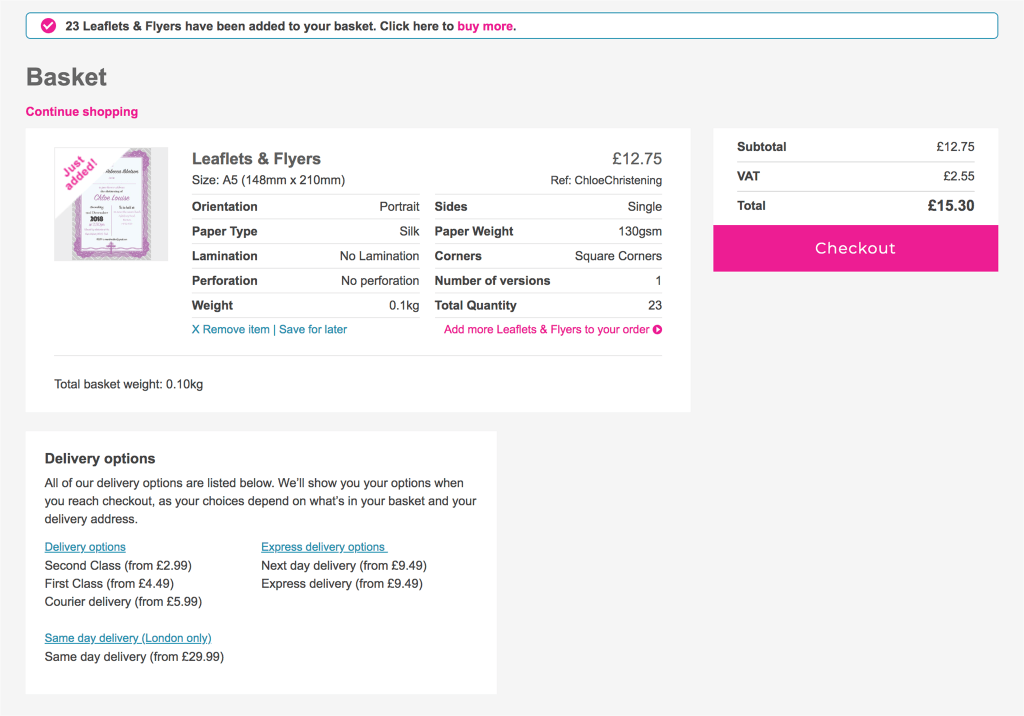Screenshot of an online shopping cart displaying a detailed view of a purchased item. The top-left corner of the screen clearly labels the cart as "Basket." The item listed within the basket is identified as "Leaflets and Flyers." The specifics of the item are meticulously detailed:

- Size: 1275 units.
- Dimensions: A5 (148 mm by 210 mm).
- Orientation: Portrait.
- Paper Type: Silk, with no lamination or perforation.
- Weight: 0.1 kg.
- Print Sides: Single-sided.
- Paper Weight: 130 GSM.
- Corners: Square.
- Version: One.
- Total Quantity: 23 items.

The total cost for all items is listed as $15.30.